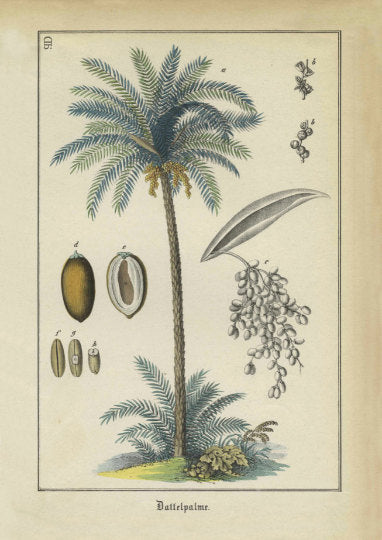This is an intricately detailed, charcoal-style yet colored drawing of a palm tree, rendered on a faded, tan parchment-like paper. The illustration, reminiscent of an ancient botany book or plant encyclopedia, is bordered by a thin black line. The tree's trunk is a muted brown, crowned by feathered leaves in varying shades of green and light green, with some yellow leaves emerging from beneath the canopy. At the base of the trunk, a small, grassy patch with green bushes adds depth and texture.

On the left side of the image, a coconut and its halved section are precisely illustrated, revealing the white meat inside. To the right, a black and white diagram details a flowering palm leaf, showcasing the intricate structure typically found below the palm fronds. At the bottom of the drawing, there is a stylized text in a Romanesque font that appears to read "Diatropome," adding a textual element to this beautiful, encyclopedic illustration.